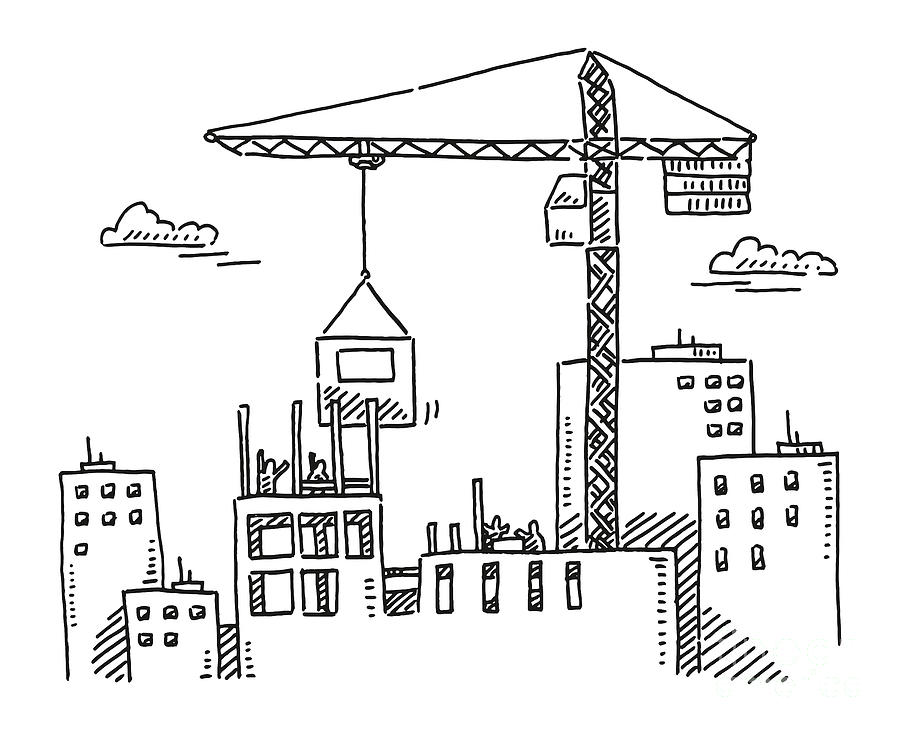This detailed pen sketch, rendered in black ink on a white background, vividly captures a bustling cityscape featuring a construction site. The scene is centered around six skyscrapers, some of which are still under construction. Two of the skyscrapers prominently feature human figures—workmen toiling away on the structures. The middle and lower sections of these buildings are particularly populated with these workers, suggesting active construction.

Dominating the right center of the sketch is a tall, narrow building crane, complete with a cab, boom, pulleys, and a counterbalancing weight. Attached to the crane is a lift cage, depicted as lowering a piece of the building onto one of the skyscrapers. The backdrop of this intricate scene is marked by two fluffy clouds, one floating on the left and another on the right, adding to the whimsical, cartoon-like artistry of the drawing.

Overall, the sketch combines technical details of urban construction with an artistic, almost caricatured style, effectively conveying a dynamic city scene in a simple yet detailed black-and-white format.